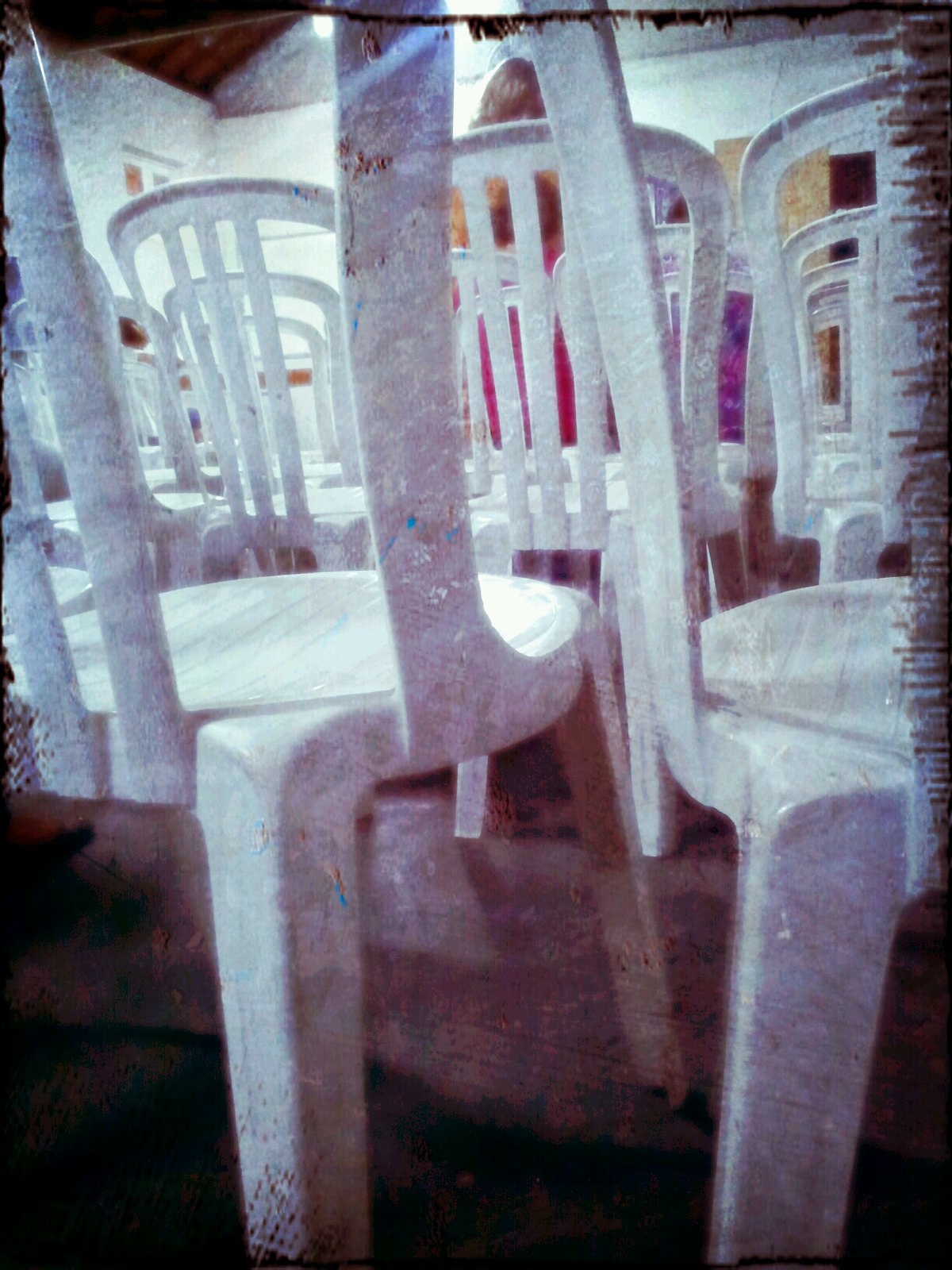The real-life photograph, with a distressed, aged feel, showcases a room filled with numerous inexpensive, white plastic patio chairs typically found at big box stores. These chairs, characterized by their textured seats and rounded backs with slats, are somewhat flimsy and shiny. The image's view is at seat level, revealing a person with long hair and a pink shirt seated three rows ahead, glimpsed through the slats of the preceding chairs. The foreground chair features some splatters of blue paint on its back. The photograph is very grainy, exhibiting grey and black patterned noise around the edges and visible degradation into dark, blank spots and visual distortion, particularly on the right side. This distortion resembles a grungy filter effect, with parts of the scene appearing scraped away as if by paint thinner. The setting includes a dark floor and white walls, with a small window on one side and a wooden door on the other. Light filters through from above, illuminating the scene under a wooden ceiling. The photograph is framed by a brown border, enhancing its vintage aesthetic.